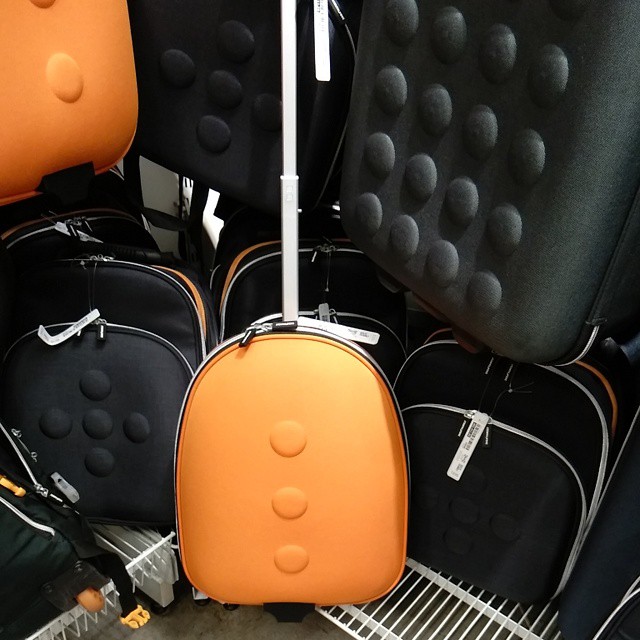The image depicts a display of various travel bags and suitcases, arranged on a white metal rack with a concrete floor beneath. The luggage is a mix of black and orange bags, some made from stiff fabric material. The black bags often feature circular studded designs, with quantities ranging from four to sixteen visible circles. An orange bag, centrally located and backpack-shaped, has three vertical dots and a pole protruding from the back, indicating it may be a roller bag. The black bags occasionally have an orange lining or piping around the zippers. Additionally, each bag bears a bar-coded tag, suggesting they are ready for travel or for sale. The arrangement includes bags both resting on a lower shelf and suspended from an upper section, with some bags showing protruding straps and belt-like clips for securing contents.